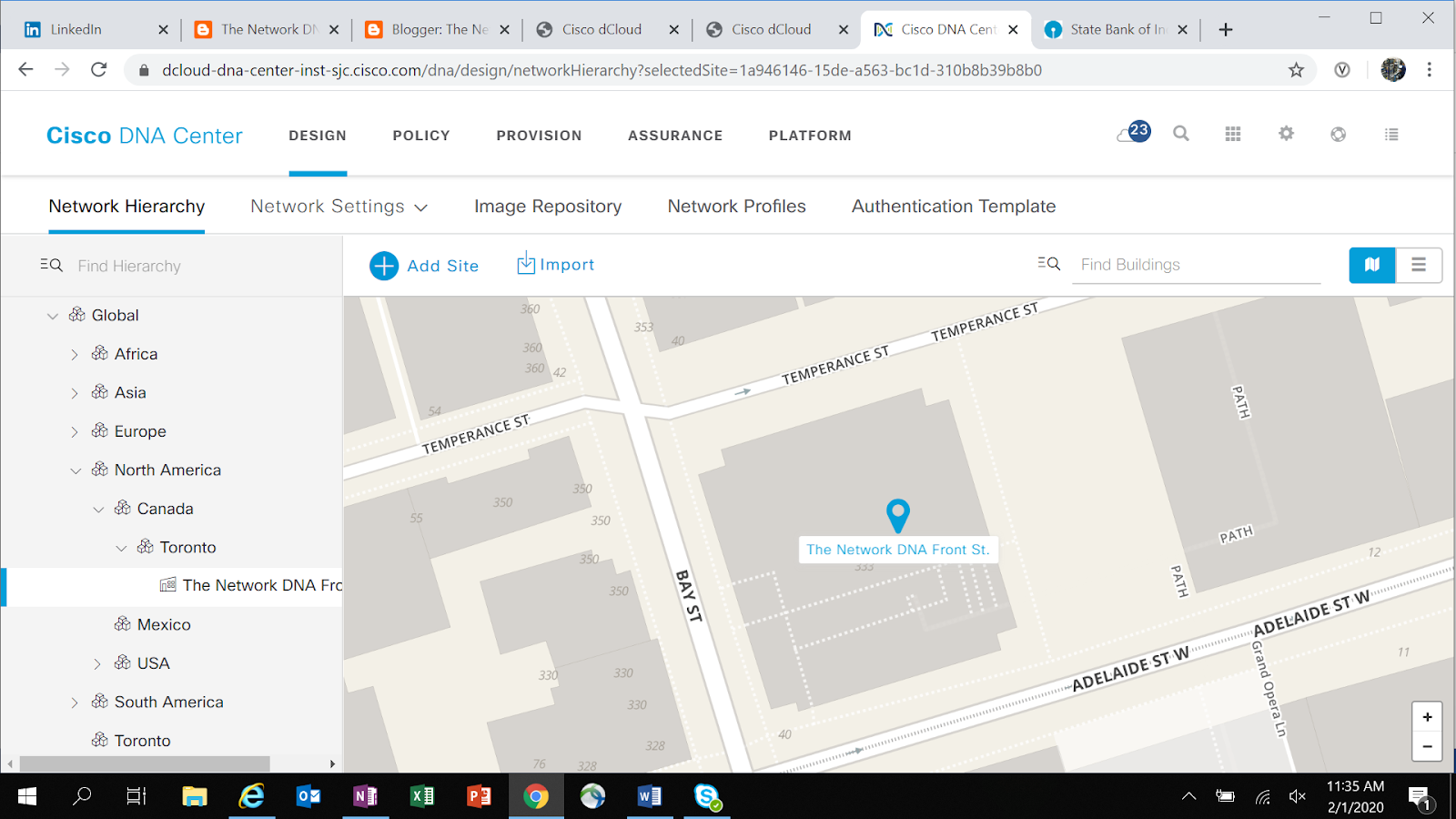Here is the refined descriptive caption for the image:

"Screenshot of a computer displaying multiple active web tabs, including LinkedIn, The Network, Blogger, Cinco Cloud, Cinco D-Cloud, and State Bank, each featuring an "X" icon for closing. At the center, the Cisco DNA Center interface is open, highlighting sections such as Design, Policy, Provision, Assurance, and Platform, with 'Design' underlined in blue. Below, Network Hierarchy is underlined in blue, followed by options like Network Settings, Image Repository, Network Profiles, and Authentication Template. A map resembling Google Maps displays an urban area with streets like Temperance Street, Bay Street, Adelaide Street West, and Front Street. A blue map symbol marks 'The Network Hierarchy' location. On the left, a sidebar lists categories and subcategories including Global, Africa, Asia, Europe, North America, with further regional breakdowns like Canada, Toronto, DNA, Mexico, USA, and South America."